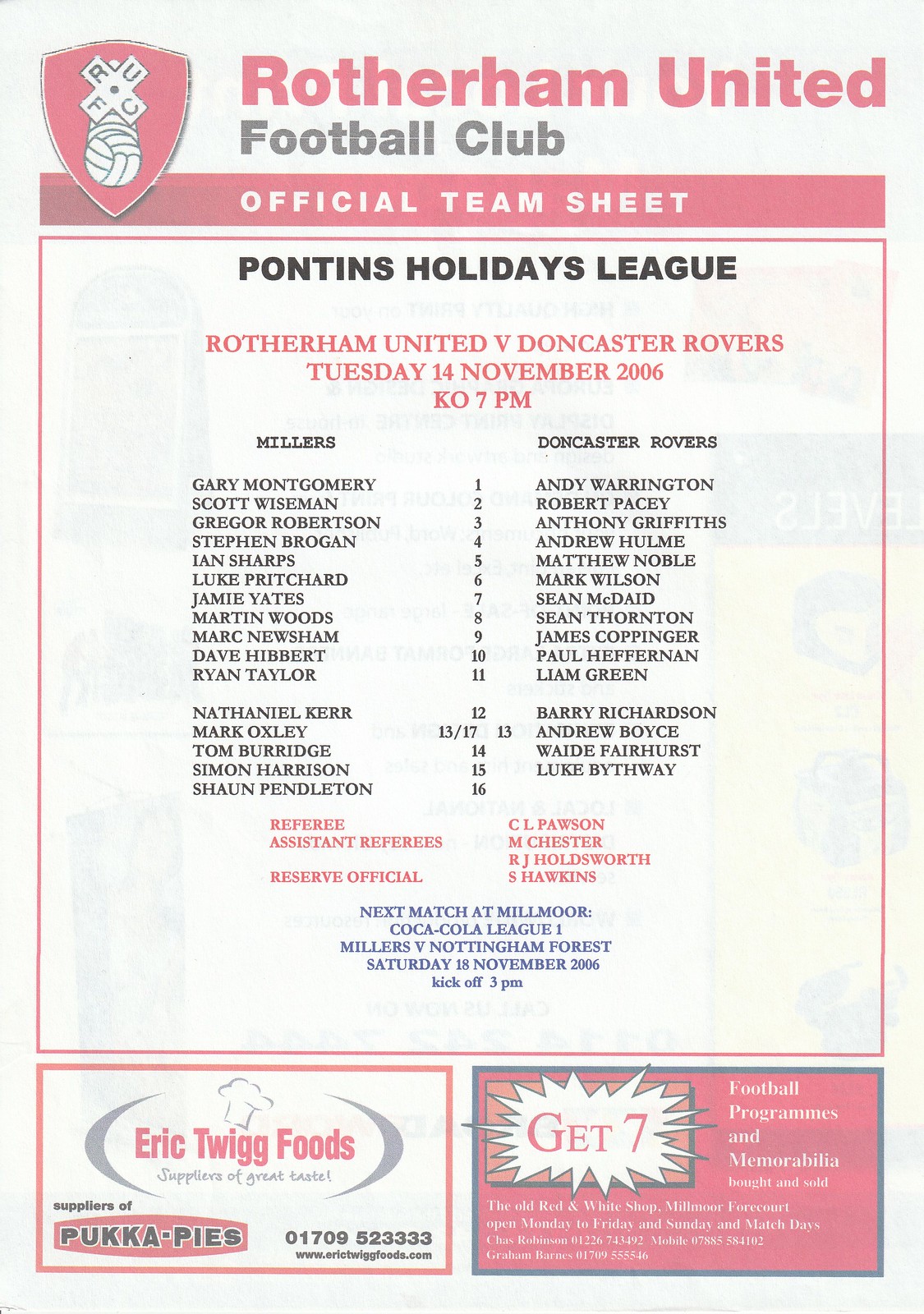This image is a scanned official team sheet of a Rotherham United Football Club match, featuring a predominantly white background with red and pink accents. At the top, the document headlines "Rotherham United Football Club," accompanied by the club’s crest—a diagonally tilted cross with the letters "RUFC" and a football beneath it. The sheet, titled "Pontins Holiday League," details a fixture: Rotherham United versus Doncaster Rovers on Tuesday, November 14, 2006, with kickoff (KO) scheduled for 7 PM.

The layout divides into two columns listing players from both teams, "Millers" (Rotherham United) on the left and "Rovers" (Doncaster Rovers) on the right. Key players for the Millers include Gary Montgomery (1), Scott Wiseman (2), Gregor Robertson (3), Ian Sharps (5), and more, totaling around 12 to 15 names with jersey numbers indicated. The sheet also provides details about referees, assistant referees, and reserve officials. Towards the bottom, the next match location is identified as Millmoor for a Coca-Cola League One game. Additional notes include sponsors such as Eric Twigg Foods and Pucca Pies on the bottom left, and information about football programs and memorabilia on the bottom right.